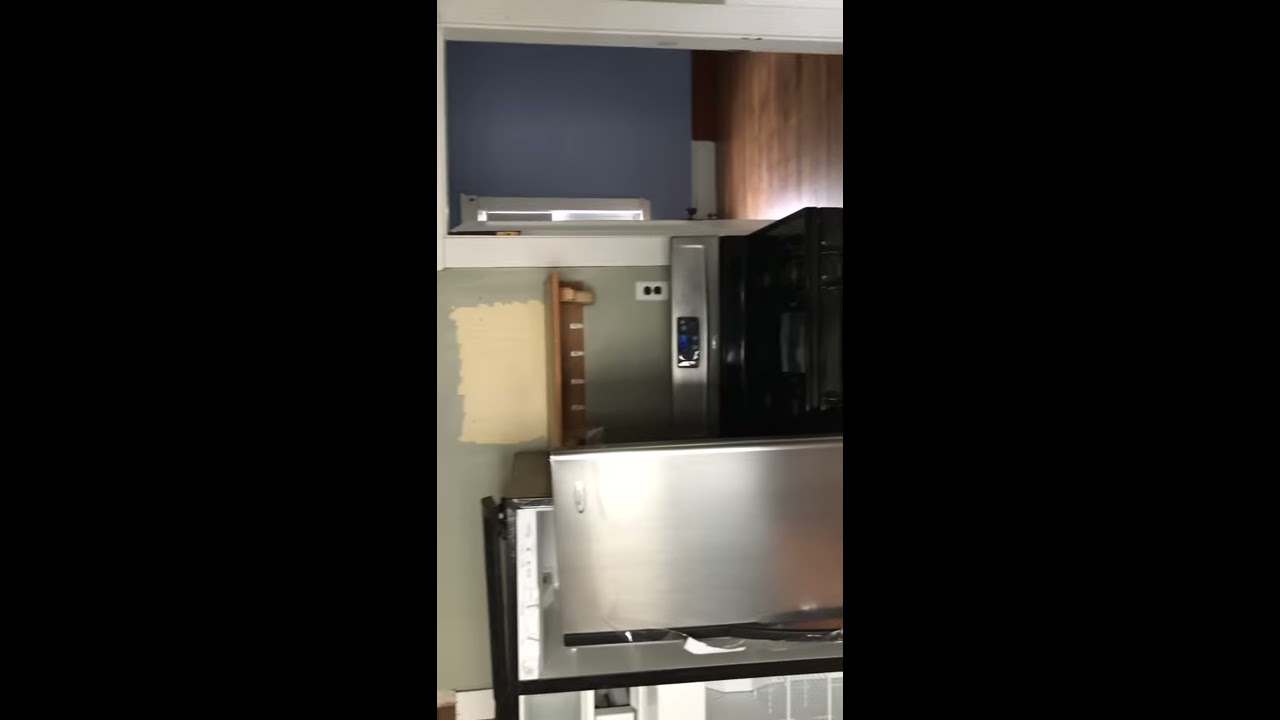In this detailed image, portrayed in portrait mode and turned 90 degrees counterclockwise, we see a section of a kitchen illuminated with indoor lighting. Dominating the lower area of the photo is a stainless steel refrigerator, its door open to reveal a glimpse of the interior. Above the refrigerator is a brown spice rack with a yellow towel hanging from it, and further up, a silver appliance that could be a microwave. To the right of the refrigerator (which would be towards the upper part in the rotated view), a white-trimmed doorway leads into an adjacent room with a blue wall and a wooden plank floor. Visible through the doorway is a window also framed with white trim, and there is an additional entryway to the left of the refrigerator suggesting another passage out of the kitchen. The background walls feature two electrical outlets beneath a wall-mounted light fixture, and there's a white cutout in the wall that appears to be a storage area. The overall scene combines elements of functional kitchen design with a hint of industrial aesthetic.